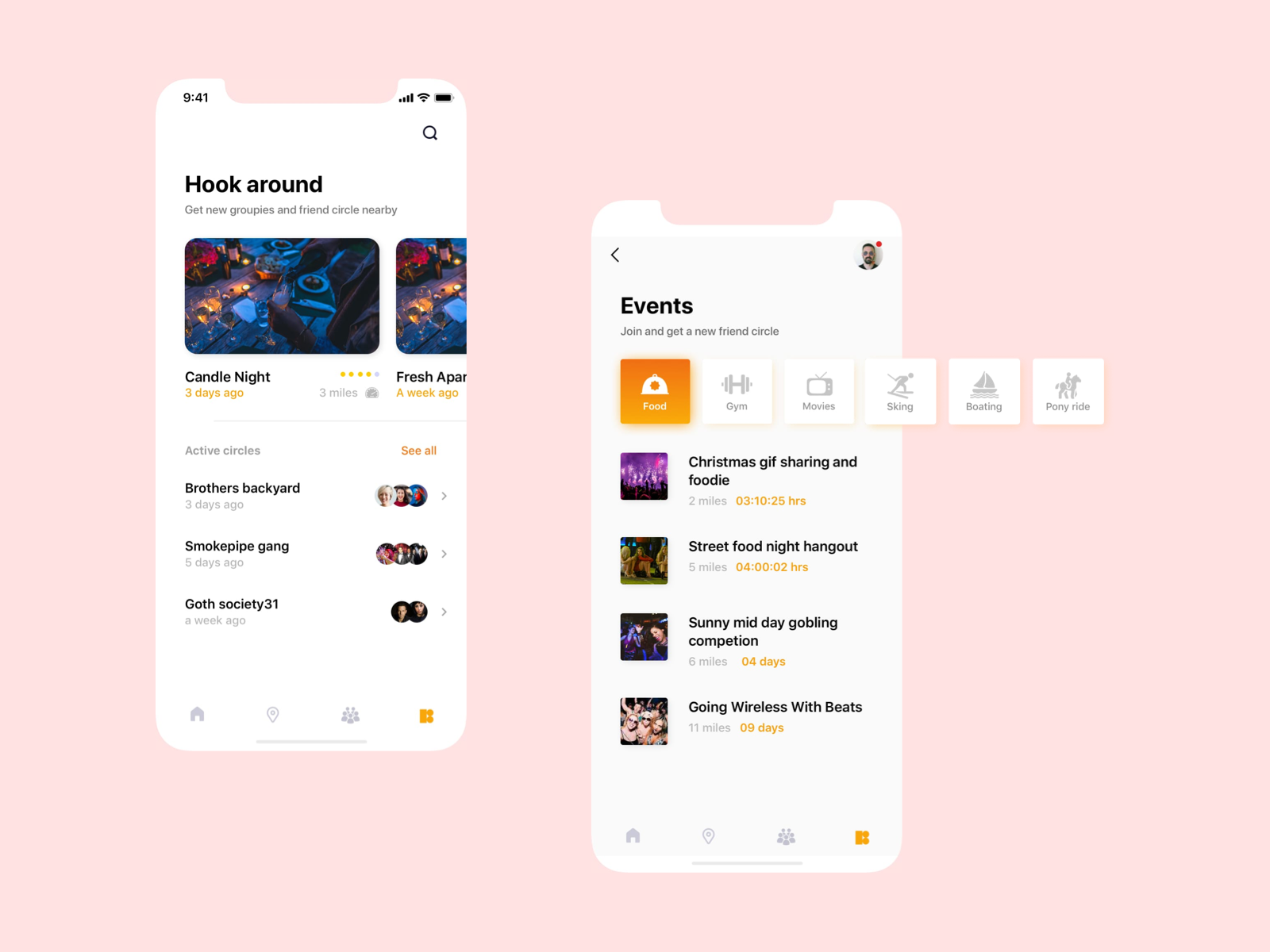This image features a vibrant pink background, centering two smartphone screenshots. 

The left screenshot displays text in bold black letters reading "Hook Around," followed by a description: "Get new groupies and friends circle nearby." Below, an image of candles on a table is accompanied by text: "Candle Night," marked as having occurred "3 days ago" and located "3 miles" away, but the rest of the text is cut off. Further down, it lists various active circles and their recent activities:
- "Brothers Backyard," with a social media thumbnail, took place "3 days ago."
- "Smoke Pipe Gang," occurred "5 days ago" with some social media images.
- "Goth Society," listed as "31" took place "a week ago."

The right screenshot, labeled "Events" at the top, encourages users to "Join and get a new friend circle." It features categories such as Food, Gym, Movies, Skiing, Boating, and Pony Rides. Below, several event descriptions appear:
- "Christmas Gift Sharing and Foodie," located "2 miles" away.
- "Street Food Night Hangout," "5 miles" away.
- "Sunny Midday Gobbling Competition," "6 miles" away.
- "Going Wireless with Beats," "11 miles" away.